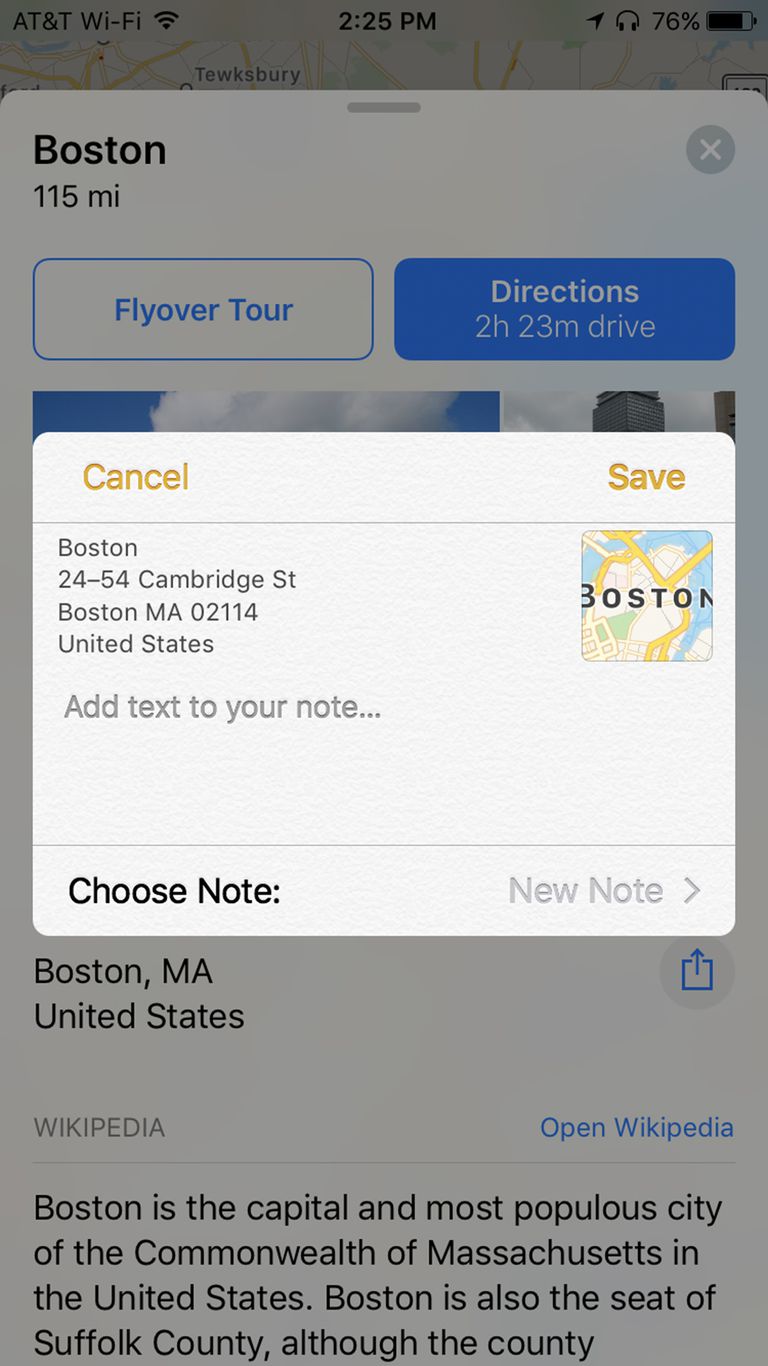In the image, a device screen is displayed showing information typical of a smartphone interface. The upper part of the screen indicates that the device is connected to AT&T Wi-Fi with full signal strength, and the current time is 2:25 PM. Additionally, an icon shows the battery level of connected Bluetooth headphones at 76%.

Prominent on the screen is a map showing Boston and its surroundings, with a blue rectangle providing directions. The text within the rectangle indicates a route towards Boston, Massachusetts, approximately 115 miles away. Specific directions within the program appear in orange text.

Further text information includes details such as the address “2454 Chemistry, Boston, Massachusetts, 02114”. A portion of this text appears to be extracted from a Wikipedia article, stating: “Boston is the capital and most populous city of the Commonwealth of Massachusetts. Boston is also the seat of Suffolk County.” The background is grey, with white text, and a central highlighted square in a lighter color, possibly indicating selected or active content.

The overall interface suggests a navigation or travel-planning application with integrated Wikipedia information for easy reference.